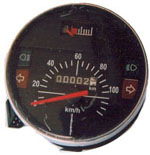This close-up image features a speedometer that has been removed from a vehicle, likely a motorcycle or a moped. The speedometer has a white, circular face displaying measurements in kilometers per hour (km/h), ranging from 0 to slightly above 100. An orange needle indicates the current speed, while a centrally located odometer shows a reading of 2 kilometers. The brand name, although partially obscured due to the small size of the photograph, is positioned at the top of the speedometer. Adjacent to the speedometer on the left are two unlit indicator lights: an orange square with a left-facing white arrow, possibly indicating a left turn signal, and a green light with an ambiguous shape, likely a blinker symbol. These indicators suggest directional signals for the vehicle.